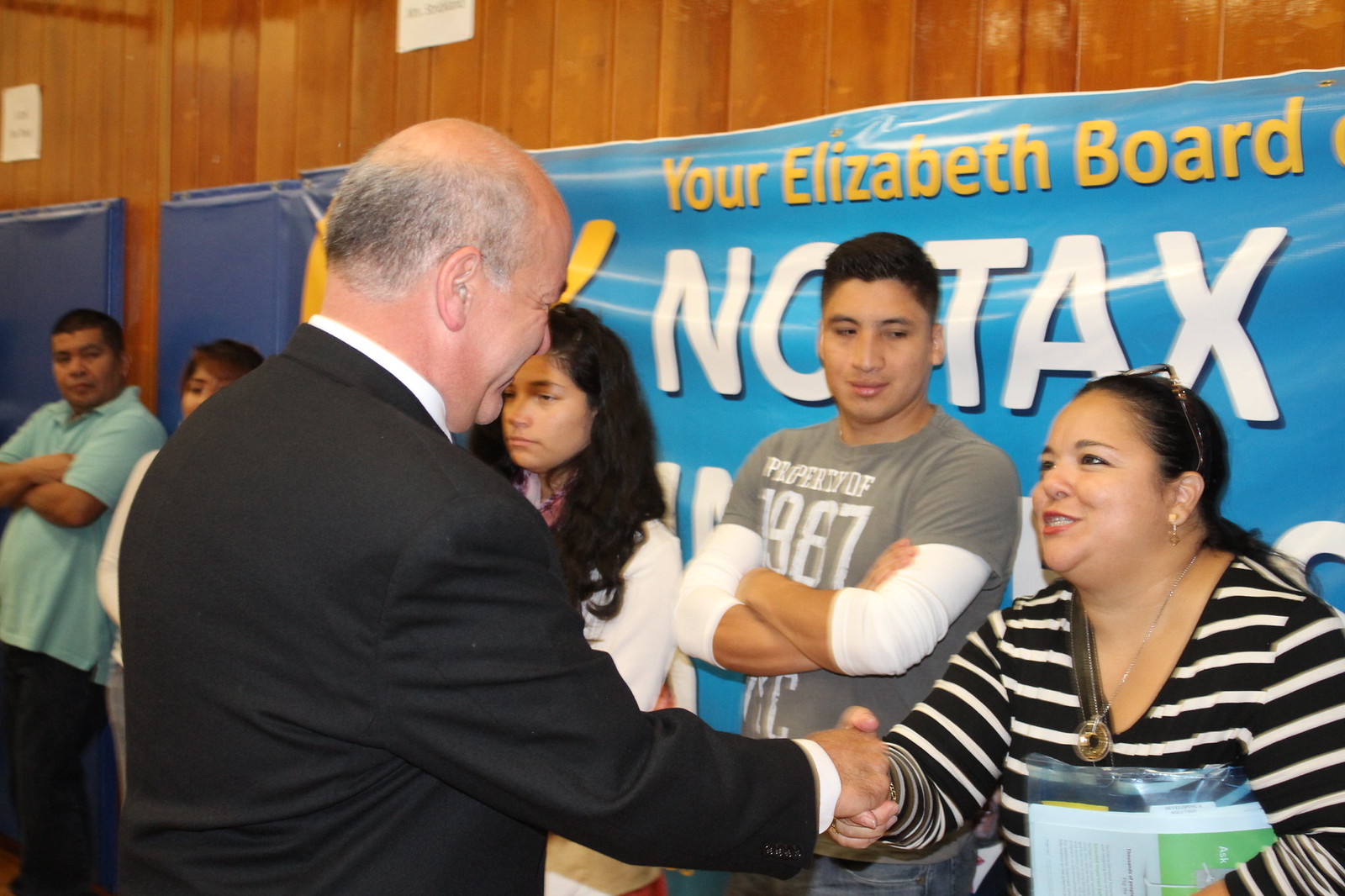In the image, a balding politician with gray hair is seen shaking hands with a woman in a black and white striped top. The politician, dressed in a black jacket and white shirt, is facing away from the camera towards the citizens. The woman, who appears to have Latin origins with a white complexion, is wearing a necklace with a circular medal pendant, silver earrings, and eyeglasses perched on top of her head. She is smiling warmly at the politician. Behind her, several other people, including women and men, stand in line, likely waiting to greet the politician. In the background, a blue banner with partially obscured text reads, "Your Elizabeth Board" and "No Tax," and is affixed to a wall made of vertical wood planks. The setting features additional blue elements in the top left corner of the image.